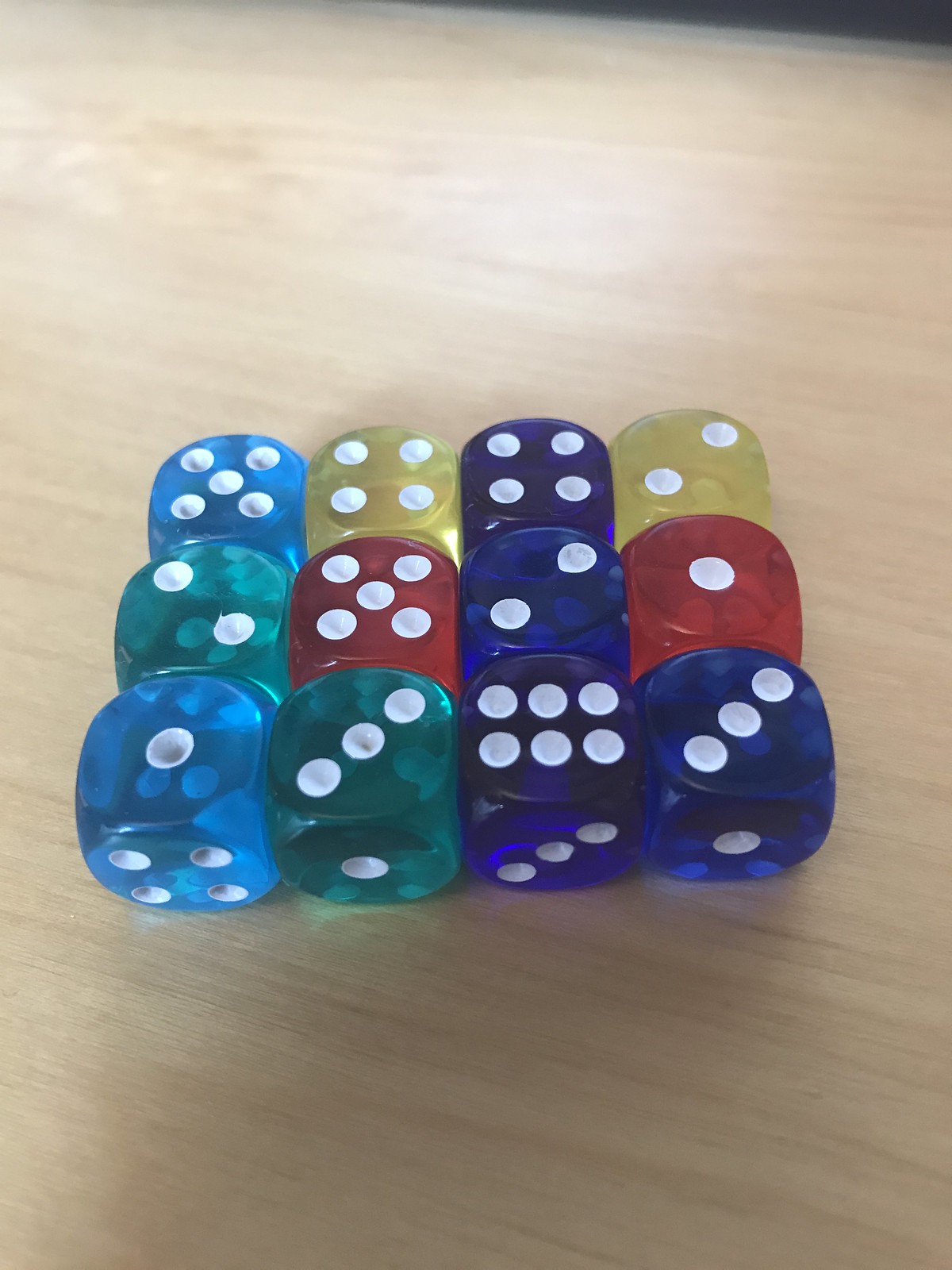In the photograph, twelve colorful dice are meticulously arranged in three rows of four on a light-colored brown tabletop. The dice, crafted from a transparent perspex plastic, radiate a vibrant, see-through hue. The collection features various colors: two yellow dice, four in a deep midnight blue, two in a rich red, two in a greenish-teal, and two in a light turquoise blue. Each die displays a unique set of dots, representing different numbers. Despite the absence of any discernible color order or pattern, the dice are neatly grouped together, possibly hinting at a recent purchase or an organized display of a new set. This intriguing array could be intended for a variety of games, far beyond the typical two dice used in gambling or poker, suggesting a long future of diverse gaming experiences.